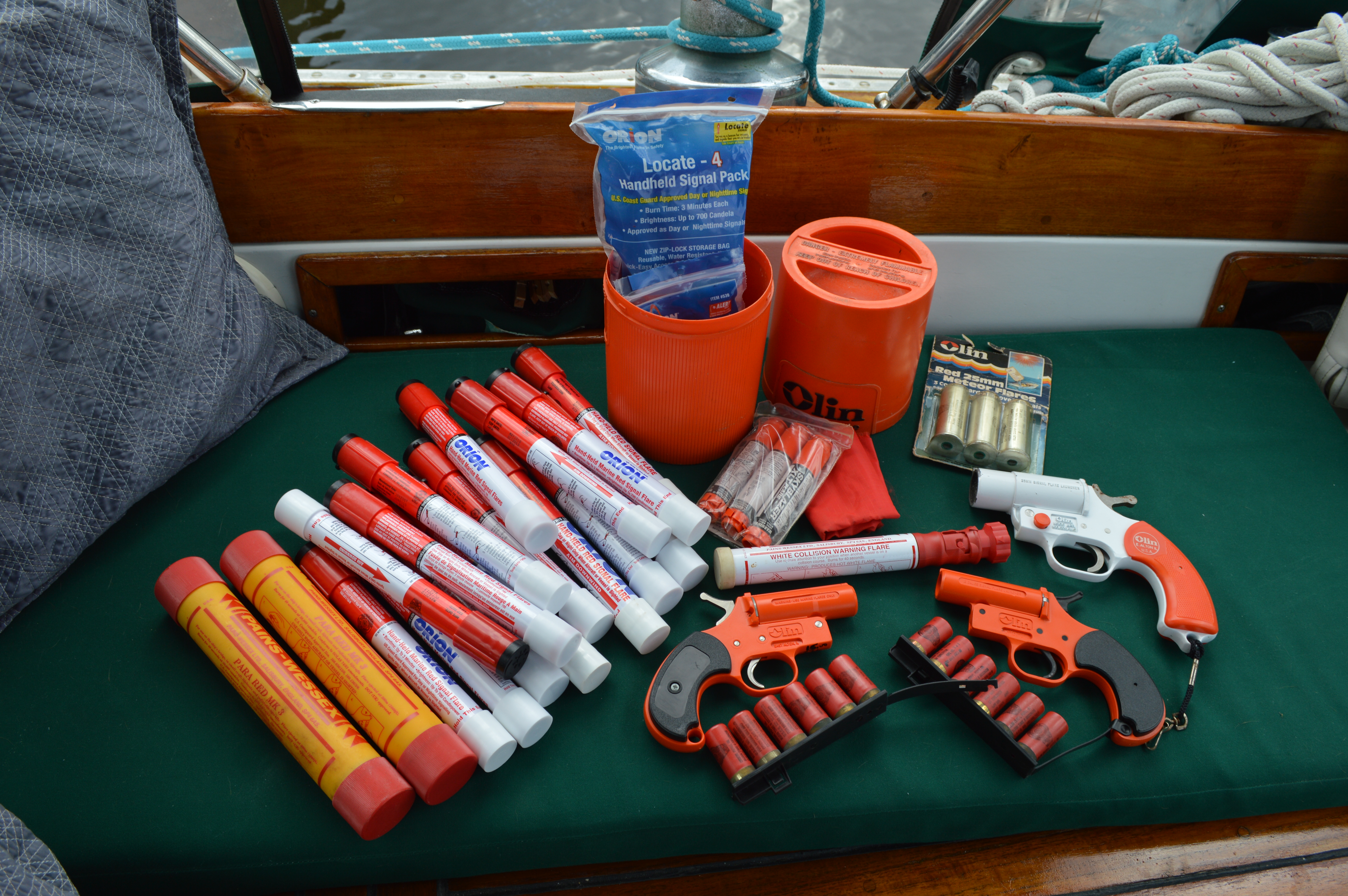This high-quality photograph captures an assortment of maritime safety equipment arranged on a green cushioned bench, likely situated on a boat. Prominently displayed are three distinct flare guns: one with a white barrel and orange handle, and two with orange barrels and black handles. Alongside the flare guns are several rounds of flare ammunition resembling small, red shotgun shells. On the left side of the bench, partially obscured, is a pillow. There is also a collection of approximately 17 variously sized flares, complete with red tops and yellow caution stickers, stored in plastic casings. Additionally, the image features orange circular containers that could be mistaken for cup holders but are likely used for storing flare-related items. The bench, adorned with wood paneling, also holds what appears to be rope, possibly tied to a pier, suggesting a nautical setting.